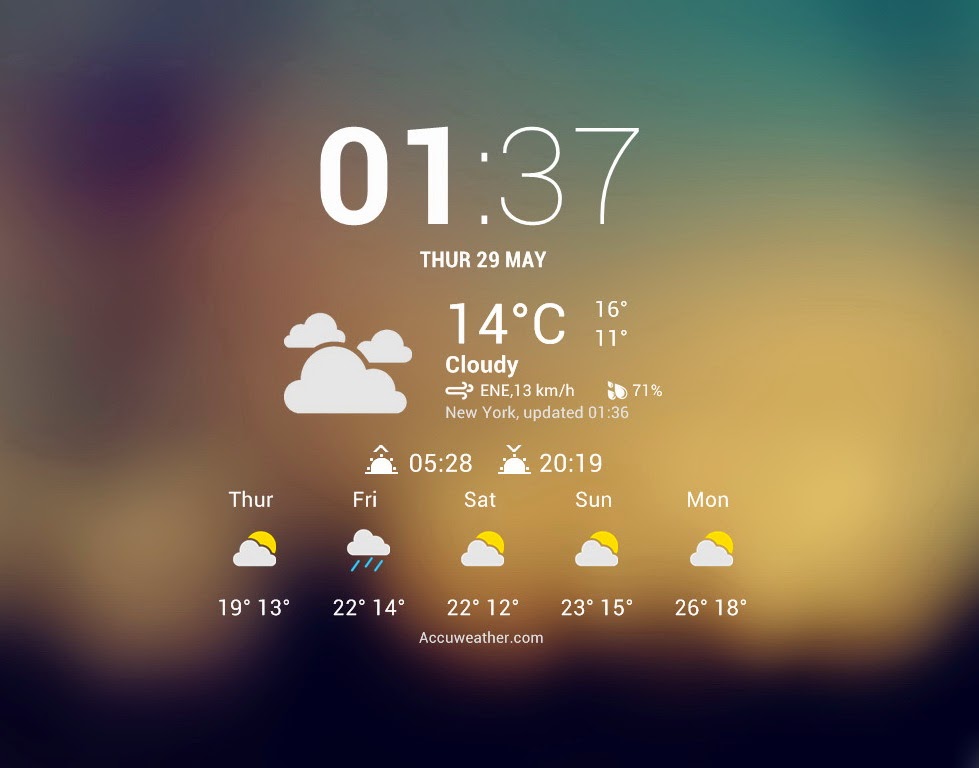A screenshot taken from a digital display showing a weather update. The background transitions smoothly from a green-teal hue in the upper right corner to purple and fuchsia shades towards the left, moving into lighter tones of orange, yellow, and tan, and finally blending into browns and then black at the bottom. The time reads 01:37, showing early morning details. The date is Thursday, 29 May, with a current temperature of 14°C and a cloudy weather description. Additional details include wind direction and speed (ENE, 13 KMH), location (New York), an update timestamp (01:36), and a temperature range for the day (high of 16°C and low of 11°C). The forecast for the next few days—Thursday through Monday—lists the daily high and low temperatures. The information sources from AccuWeather.com.